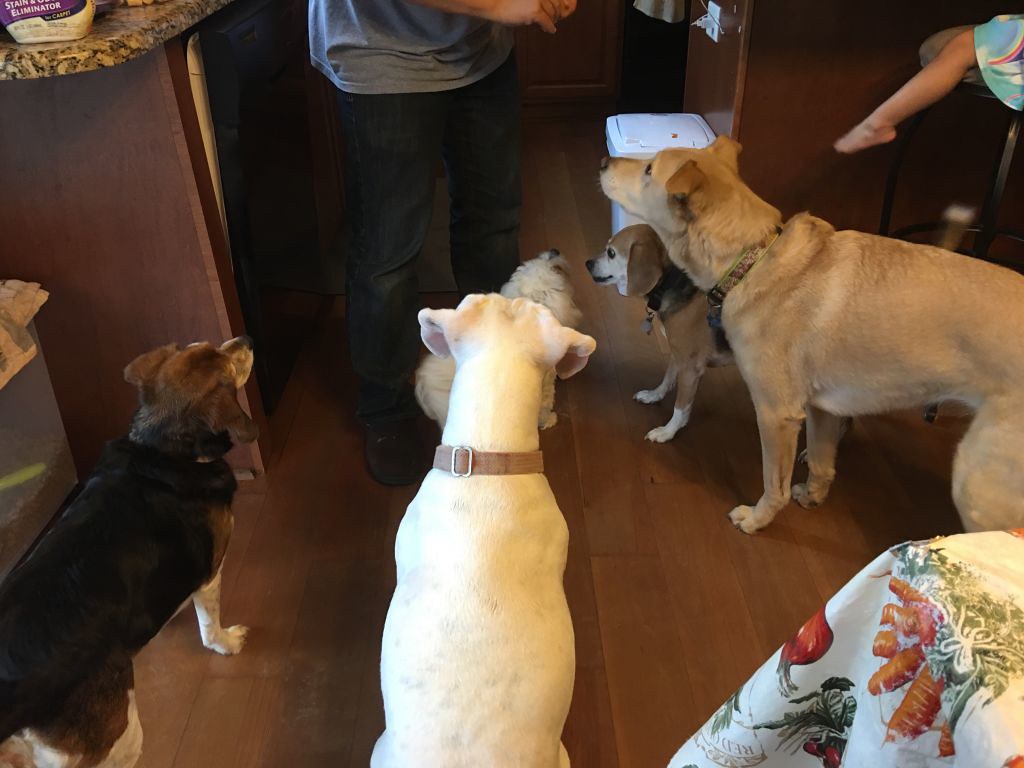The color photograph captures a dynamic scene in a kitchen, filled with attentive dogs of various breeds and sizes. Centered on the dark oak floor, a white dog with light brown patches on its ears and a brown collar with a silver buckle sits, partially cropped at the bottom. To its left stands a beagle, distinguished by its black body, brown head, and white paws. Adjacent to the beagle is another smaller beagle further from the camera, and in front of the sitting white dog is a small white poodle. On the right side, a large, tan Alsatian-type dog with darker ears stands in profile, alongside a yellow Labrador facing slightly left.

All the dogs are focused on a person whose lower half is visible. Clad in black pants and a gray shirt, the individual, likely engaging the dogs with treats or attention, immerses the scene in anticipation. The kitchen itself features dark brown oak cabinets and a yellow marble countertop with noticeable black wavy details, framing the left portion of the image. Additionally, a child's leg, likely seated on a stool, and a woman's leg, crossing from the upper right, hint at more people present. The hardwood floorboards run from the back to the front, accentuating the cozy and lively kitchen atmosphere.